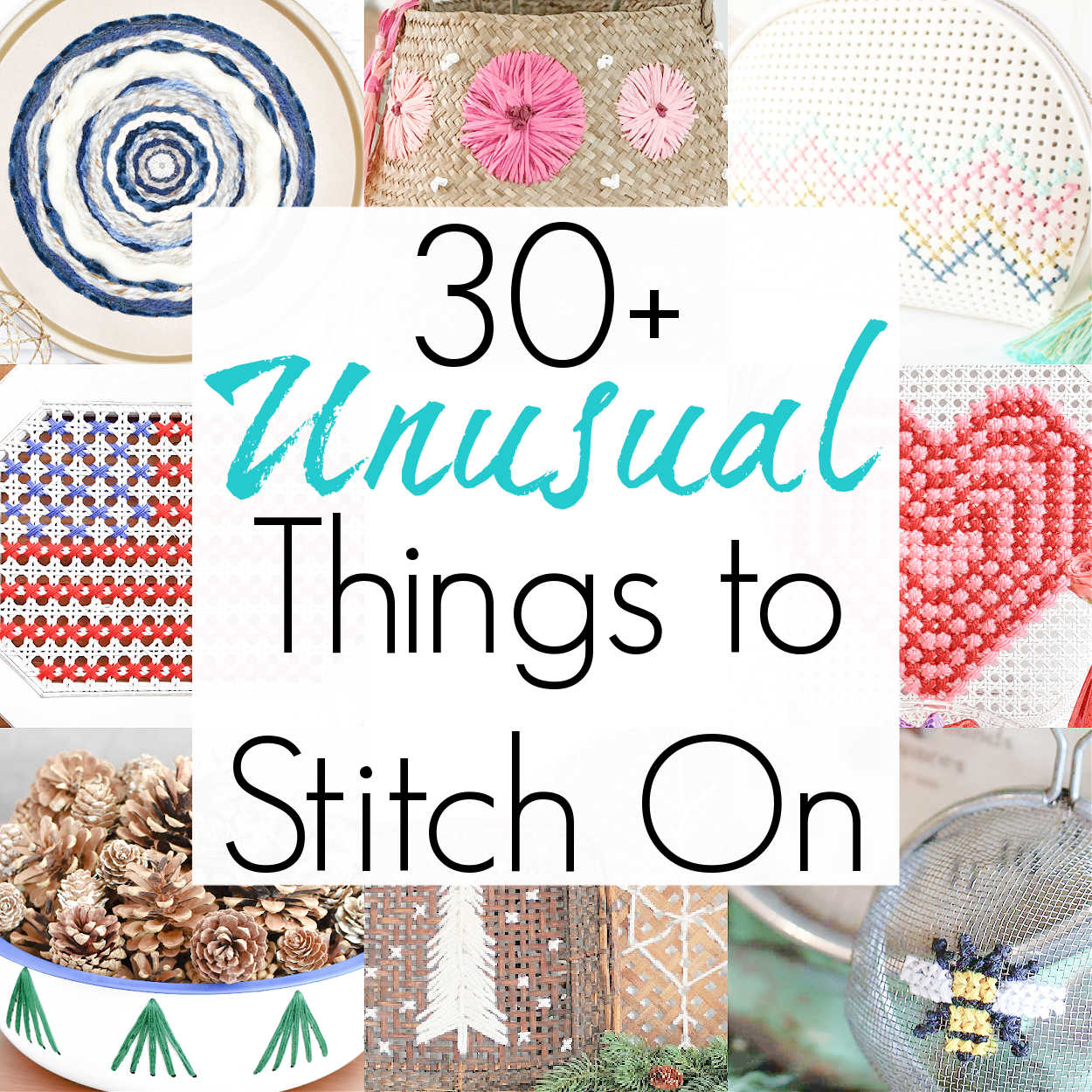The image appears to be an advertisement or cover for an arts and crafts book, prominently featuring the text "30+ Unusual Things to Stitch On" in the top-center white square. This main title employs a cursive, blue crayon-like font for the word "unusual," while the rest of the text is in standard computer font. Surrounding the central text are eight distinct images organized around the square: 
1. Top left: A mix of white and blue rings.
2. Center top: A paper bag decorated with pinkish flowers.
3. Top right: A white circle with dots connected by a string.
4. Middle left: An American flag design.
5. Middle right: A heart pattern.
6. Bottom left: Pine cones in a cup.
7. Bottom center: A stitched white Christmas tree and snowflake.
8. Bottom right: A bee on a colander.

Each image showcases various artistic projects, emphasizing the range of creative and unusual surfaces suitable for stitching projects.